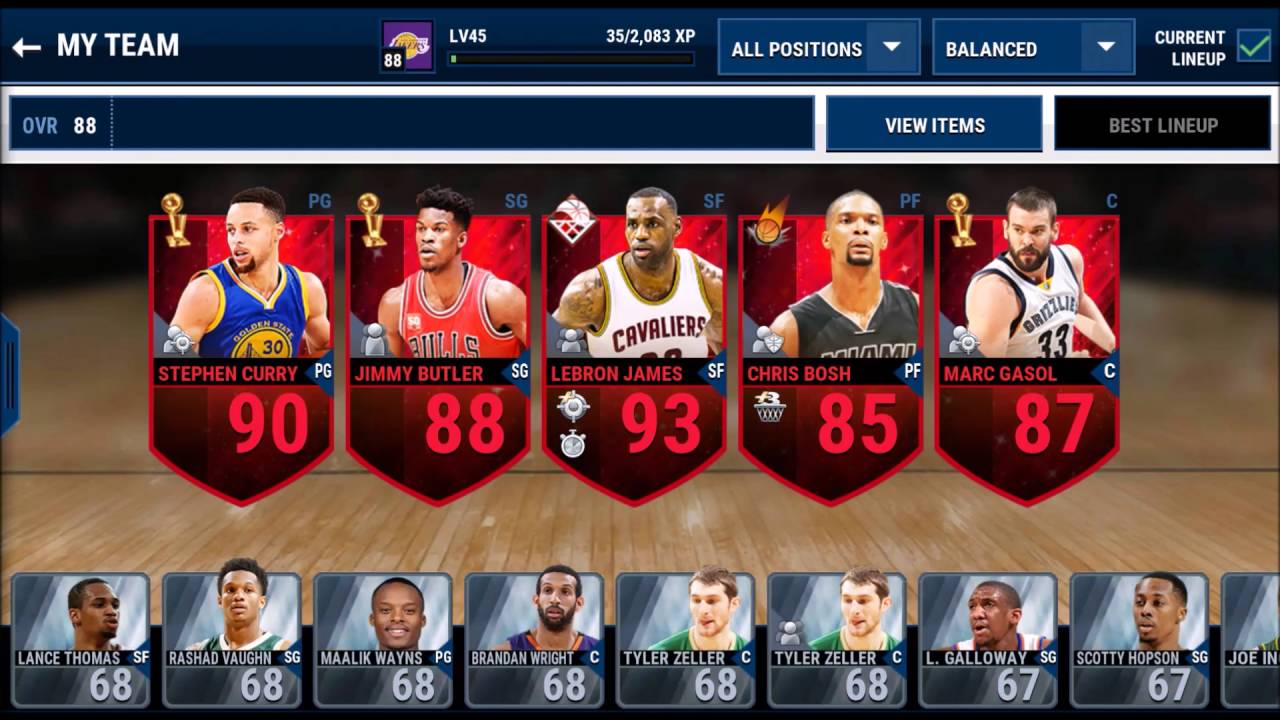Here's a cleaned-up and detailed caption for the image:

---

This image is a horizontally oriented screenshot from a PC or tablet, depicting a fantasy basketball team's interface. At the top, a dark blue banner spans almost the entire width of the page, with "My Team" prominently displayed in white on the left. In the middle of this banner, set against a navy blue background, is a small icon featuring "88 LV45" and assorted basketball-related figures.

On the right end of this banner is a light blue dropdown menu labeled "All Positions," followed by another dropdown menu labeled "Balanced." Below these menus is a section titled "Current Lineup," printed in white, next to a checked checkbox.

The subsequent part of the layout includes a thin white border line followed by another dark blue bar. Below this line is a somewhat overlapping section with options "View Items" placed under "All Positions" and partially under "Balanced," and a "Best Lineup" button in black.

Prominently displayed beneath these options are five player cards with red backgrounds, shaped like shields ending in downward arrows. Each card features the player's name, photo, and rating in red. From left to right, the players are Stephen Curry (90), Jimmy Butler (88), LeBron James (93), Chris Bosh (85), and Marc Gasol (87). All players are young black men, except Marc Gasol, who is white and positioned furthest to the right.

The bottom section is populated with smaller, square images of other players on a gray background, bearing lower ratings, typically ranging from 67 to 68. The backdrop of the player cards features an image resembling a wooden basketball court floor.